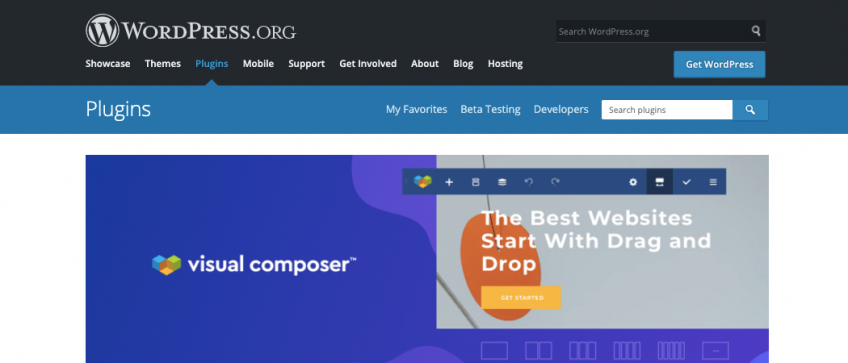The image is a detailed screenshot of the WordPress.org website. At the very top left corner, the WordPress.org logo is prominently displayed. To the right, there's a search bar labeled "Search WordPress.org." Below this, a blue button labeled "Get WordPress" invites users to download the platform.

On the left side of the page, a vertical navigation menu lists several options: "Showcase," "Themes," "Plugins," "Mobile," "Support," "Get Involved," "About," "Blog," and "Hosting." The "Plugins" tab is highlighted in blue, indicating it is the currently selected section, while the other tabs are white.

Beneath the navigation menu, the word "Plugins" is displayed again, reinforcing the chosen section. On the right side of the page, additional menu items include "My Favorites," "Beta Testing," and "Developers." 

Further into the main content area, there's a section titled "Visual Composer" with a tagline beneath it stating, "The Best Websites Start with Drag and Drop." This suggests a focus on a popular plugin that emphasizes ease of website creation through a user-friendly drag-and-drop interface.